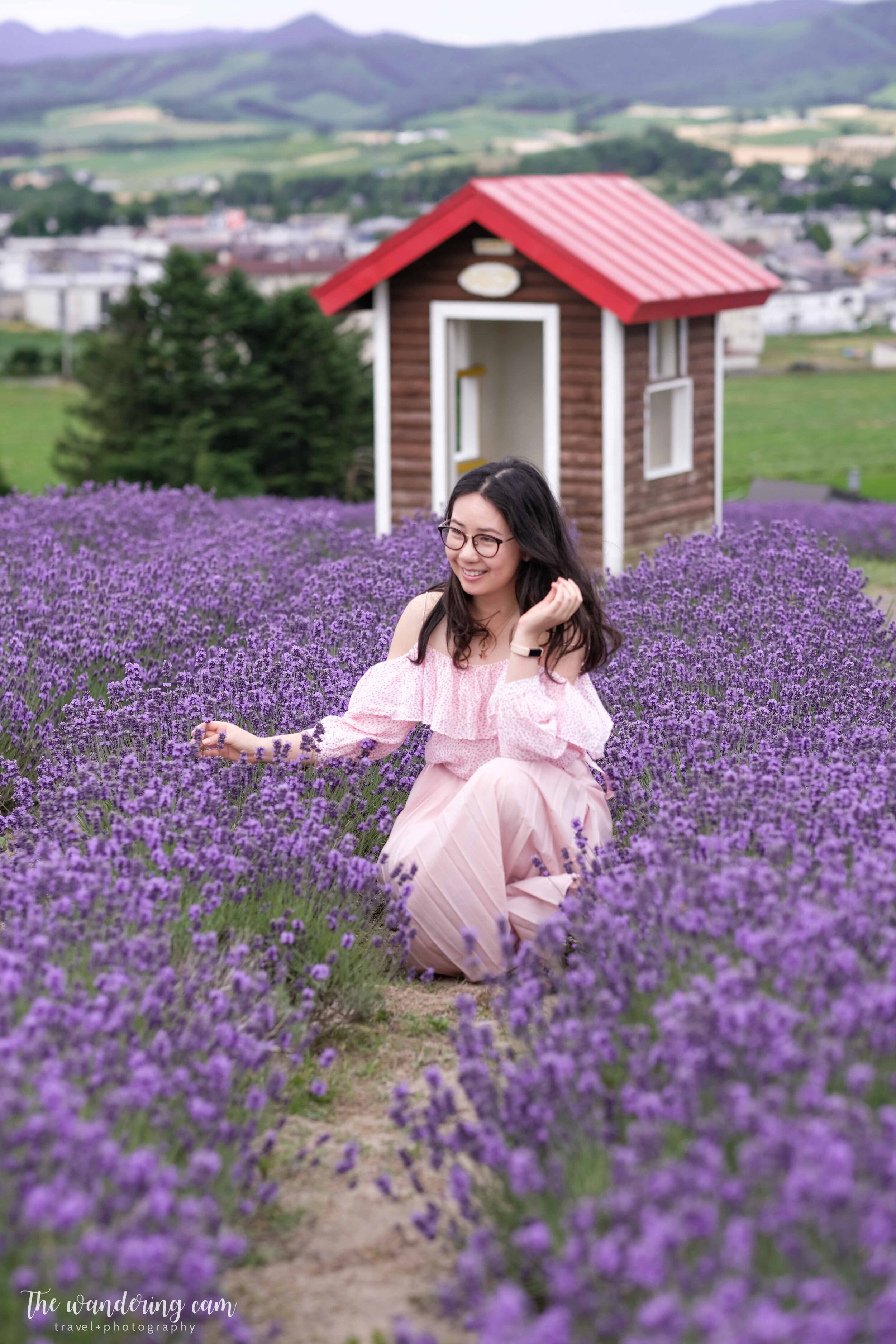In this professional outdoor photograph, a young Asian woman kneels in a dense field of vibrant purple lavender flowers, which feature green stems interspersed with rows of light brown dirt pathways. She wears a light pink, flowy dress and black-rimmed glasses, and her long, dark hair is parted down the middle, cascading past her shoulders. A pink fitness watch with a small black rectangular face adorns her wrist. She is smiling warmly, her right hand gently touching the lavender, while her left hand rests on her knee. Behind her stands a small, picturesque wooden hut with a red A-frame metal roof and white accents around the door and windows, constructed from horizontal brown wooden logs. Further back, the scene transitions into greener fields and trees, leading to the distant, blurry outline of a village with white buildings. Majestic, tree-covered mountains rise in the background, adding depth to the idyllic setting. The bottom left of the image contains text that reads, "The Wandering Cam," likely a reference to travel photography.